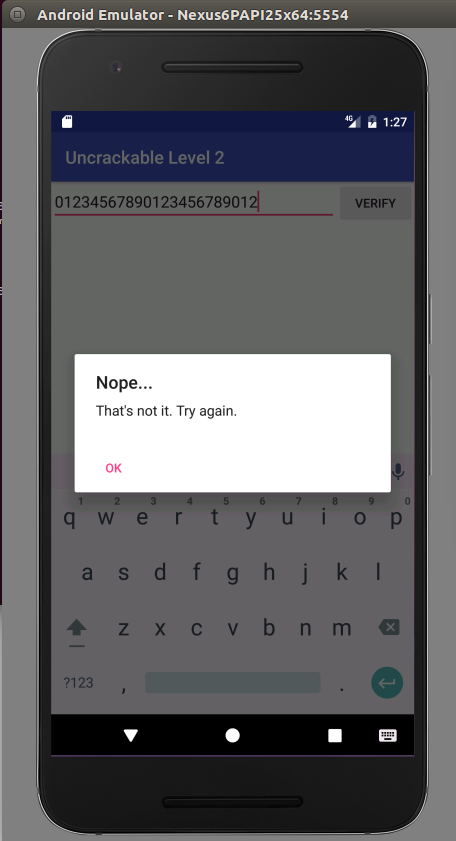The image displays an Android emulator, specifically on a Nexus device, with a large identifier number at the top. The central focus is a pop-up message that stands out against a grayed-out background, emphasizing its importance. This pop-up reads, "Nope, that's not it. Try again," and features an "OK" button for acknowledgment. Above the pop-up, the emulator showcases the title "Uncrackable Level 2," suggesting a challenge or puzzle that needs solving. Below the pop-up is a detailed number, likely related to the verification process.

The Android interface also displays a keyboard, reminiscent of the iPhone’s, capable of converting letters to numbers for input. The time on the emulator screen is shown as 1:27, accompanied by the standard array of Android status icons along the top. The overall background image appears gray, ensuring the pop-up message captures the viewer's attention. The scene implies an interactive element where the user must continue to attempt to solve the challenge by pressing "OK" and trying again, underscoring the trial-and-error nature of the task.